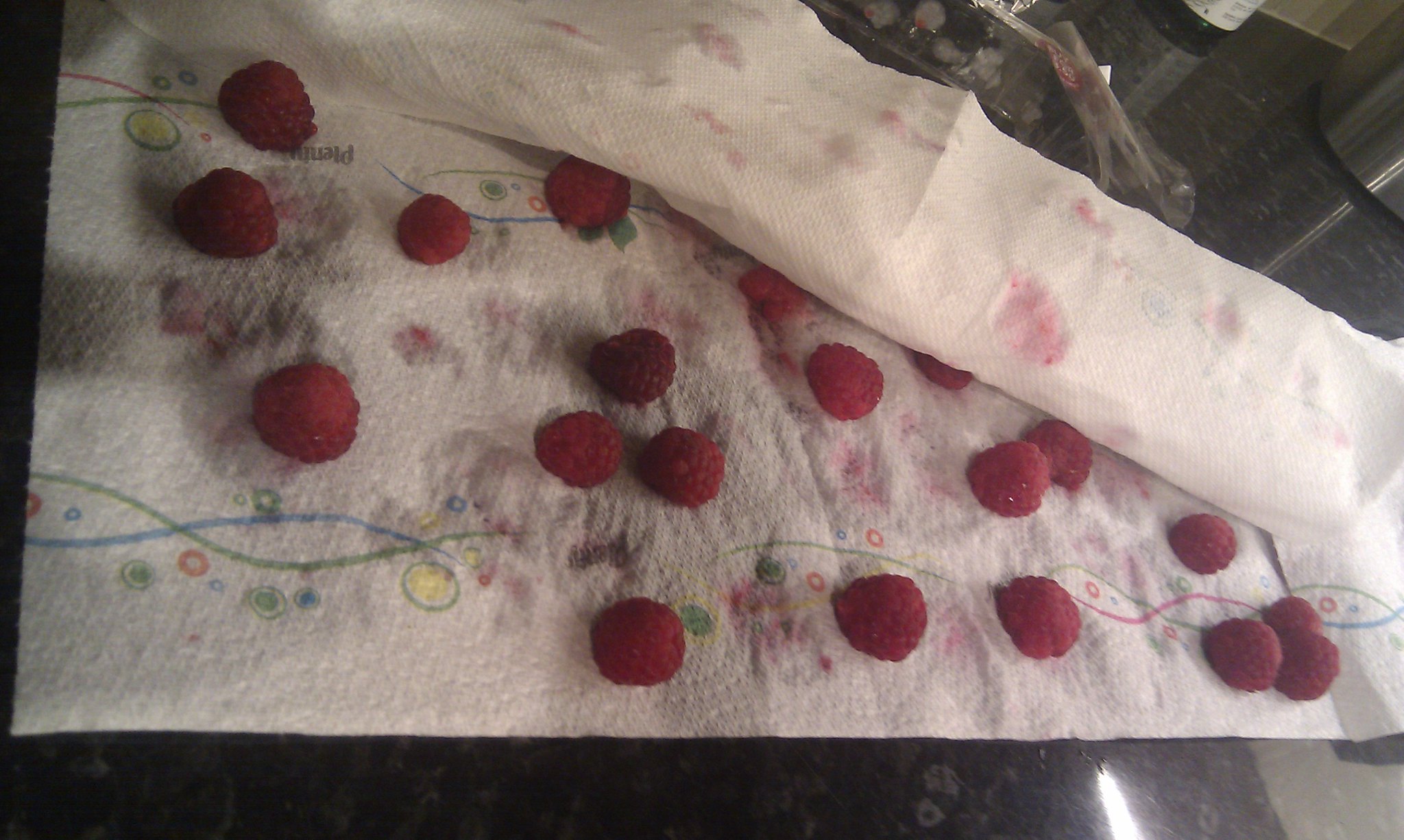The photograph depicts around twenty recently washed, vibrant red raspberries spread out to dry on a decorative white paper towel that features colorful accents in green, yellow, blue, and pink. The paper towel, which appears to be torn from a larger roll, is laid out on a black granite countertop and is partially folded over some of the raspberries, creating a blotting effect. The absorption of moisture from the raspberries has resulted in red stains and damp patches across the paper towel. Additional kitchen items, including salt and pepper shakers, are visible in the background. The raspberries are stemless, ripe, and ready to eat.